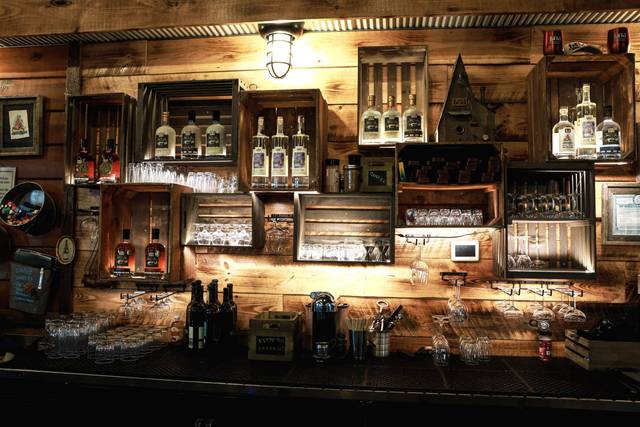The photograph captures the interior of a wooden bar, featuring a light brown wood-paneled wall and slightly darker wooden shelves that house an array of liquor bottles. The bar top is lined with several inverted glasses of various sizes and shapes, crates, and scattered shot glasses and glass containers. The shelves, stretching across the background, display rows of liquor bottles that transition in color from amber with black labels on the left to clear and white with black and white labels on the right. The bar is well-lit, with a primary overhead light and additional lighting beneath the shelves, casting a warm, yellowish glow over the scene. The central focus of the image is the bar itself, with its array of glasses and bottles, while the background shelves contribute to the rich detail of this cozy, inviting bar environment.